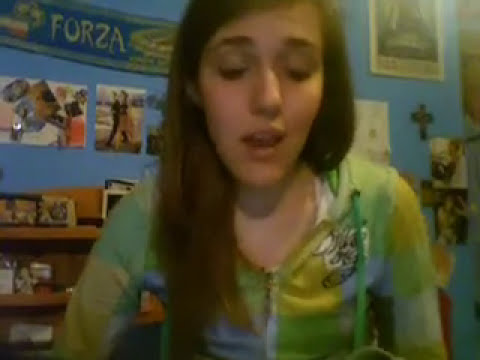A close-up, slightly blurry photo of a young Caucasian woman with long brown hair cascading over her left shoulder and tucked behind her neck on the right side. She appears to be mid-sentence, her mouth slightly open, with her eyes closed as though in the midst of blinking. She wears a long-sleeved zip-up shirt with a mix of green, yellow, and blue colors, featuring a drawstring on the right shoulder. The background is a blue wall adorned with various artifacts. On the right side of the wall, a solitary cross is prominently displayed. To the left side, a blue banner with the word "FORZA" in white letters hangs in the top corner. Below the banner are several photographs, securing a part of the wooden-colored, three-tiered shelf filled with knickknacks and photos.